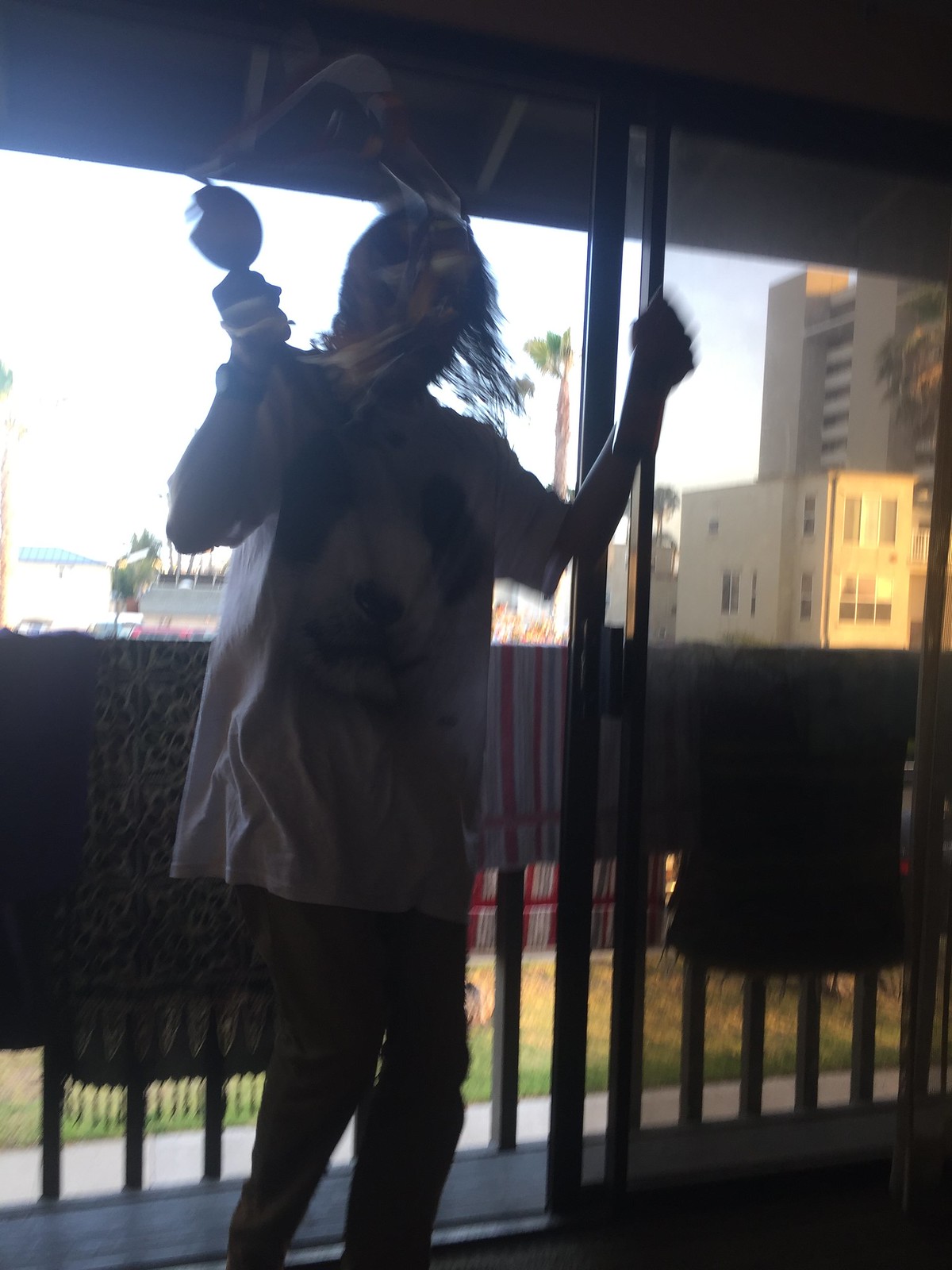A woman with flowing, shoulder-length dark hair stands on a balcony as the sun sets, casting a warm glow on a nearby apartment building seen to the right. She wears a white, short-sleeved T-shirt with a panda face design and tan pants. Both of her arms are raised near her head, as if dancing. In her right hand, she holds a maraca, while her left hand appears empty. Behind her, a sliding glass door opens onto a railing draped with a variety of colorful rugs. The scene suggests a tropical setting, with palm trees and possibly a glimpse of the ocean in the background. The overall atmosphere is slightly shadowed, likely due to the indoor lighting contrasting with the bright sunset outside.